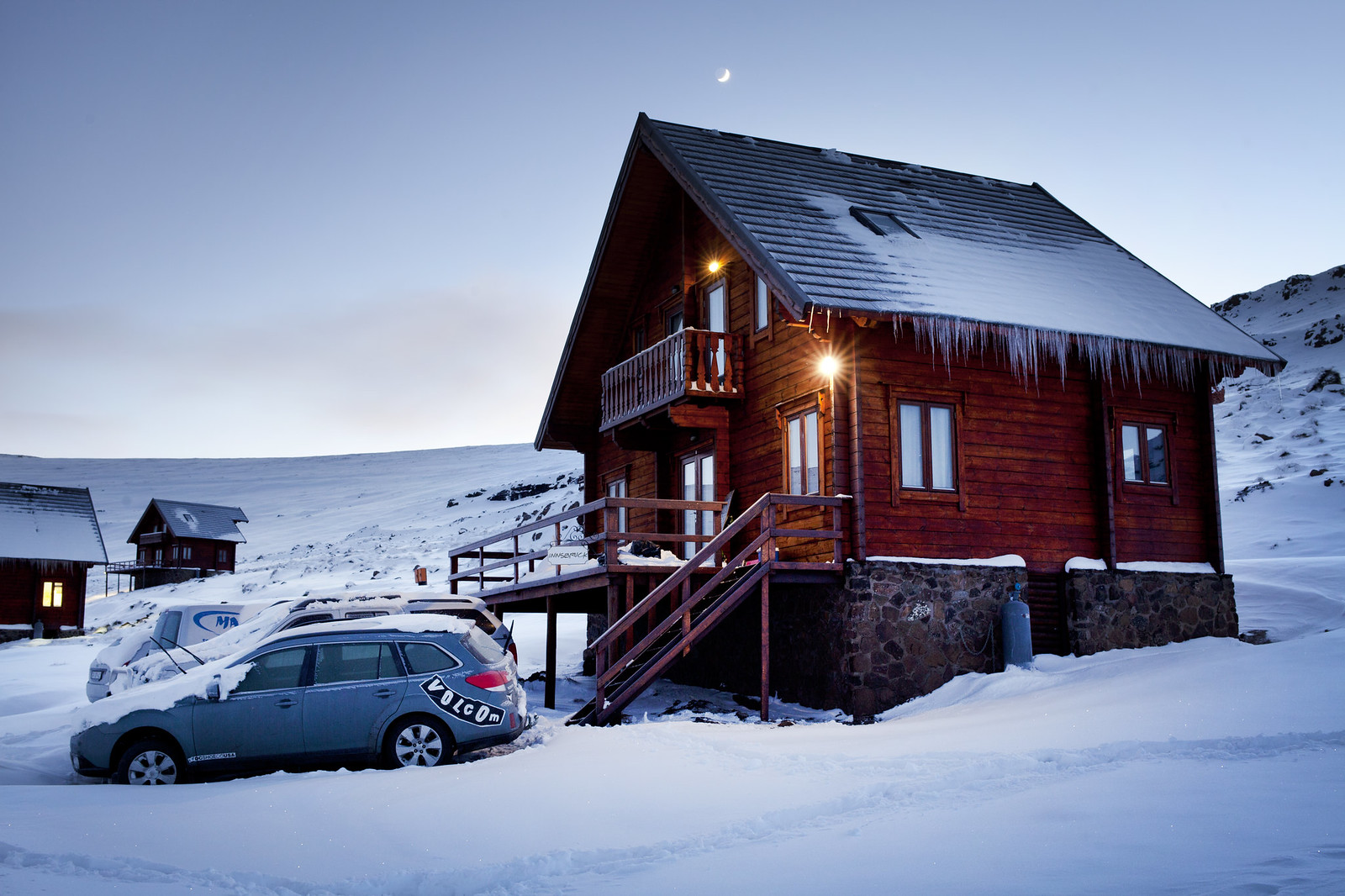Nestled against a picturesque mountain range, this charming ski chalet exudes rustic elegance and coziness. The chalet's sturdy foundation is constructed from stones and concrete, elevating the house above the ground and leading up to it via a set of quaint stairs. Clad in wooden siding, the structure features rectangular windows that allow ample natural light to filter in. 

Icicles dangle from the eaves, adding to the winter wonderland aesthetic, while a prominent skylight punctuates the roof. A sliding glass door serves as the main entrance, opening onto a welcoming deck. Upstairs, a small yet inviting balcony is tucked under the extended roofline, providing a sheltered outdoor retreat.

The chalet is warmly illuminated by exterior lights, their glow reflecting off the freshly fallen snow that blankets the surroundings. In front of the house, two cars sit, dusted with snow, hinting at a recent snowfall. The driveway, recently plowed, hints at the consistent accumulation of snow typical in this area. Flanking this charming abode are two similar ski chalets, completing the idyllic scene of this quaint mountain escape.